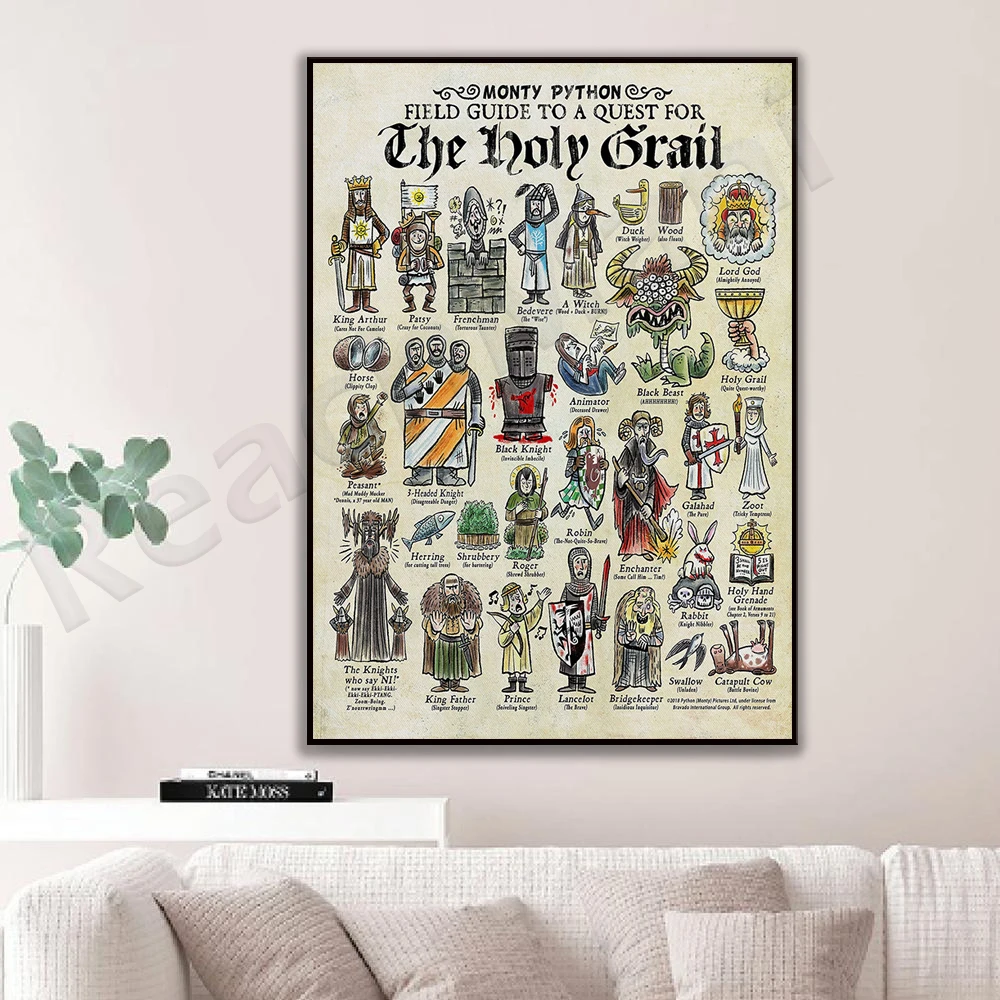The image captures a section of a living room with a focus on a framed poster and some decor elements. The off-white wall serves as a backdrop to a white couch adorned with off-white and beige throw pillows. Behind the couch is a white table with a black book titled "Kate Moss" and another white book. To the left, there is a white vase containing green leafy plants. Dominating the scene, a large rectangular poster hangs in a black frame. The top of the poster reads "Monty Python: Field Guide to a Quest for the Holy Grail" in black letters. The poster features various illustrated figures related to medieval knights and elements from the movie "Monty Python and the Holy Grail," including names like King Arthur, Patsy, Frenchman, and many others. The poster’s background is white, covered with these detailed illustrations and captions, evoking the humorous style of the movie.